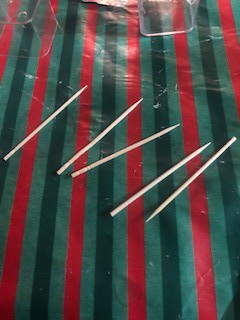This photograph features a close-up of a striped tablecloth covered surface, displaying a pattern of alternating bright red, light green, and dark green stripes that evoke a watermelon-like appearance. Resting on the tablecloth are five slender, wooden sticks, resembling either pencils or toothpicks, each with a pointed end and small ridges near their flat ends. Four of these sticks have their pointed ends directed diagonally toward the upper right, while the fifth stick's point is oriented towards the lower left. Additionally, the background includes objects cut off by the photograph's top edge, possibly identified as two clear acrylic, tube-shaped containers tipped over. The image also captures a slight reflection, indicating illumination from above.